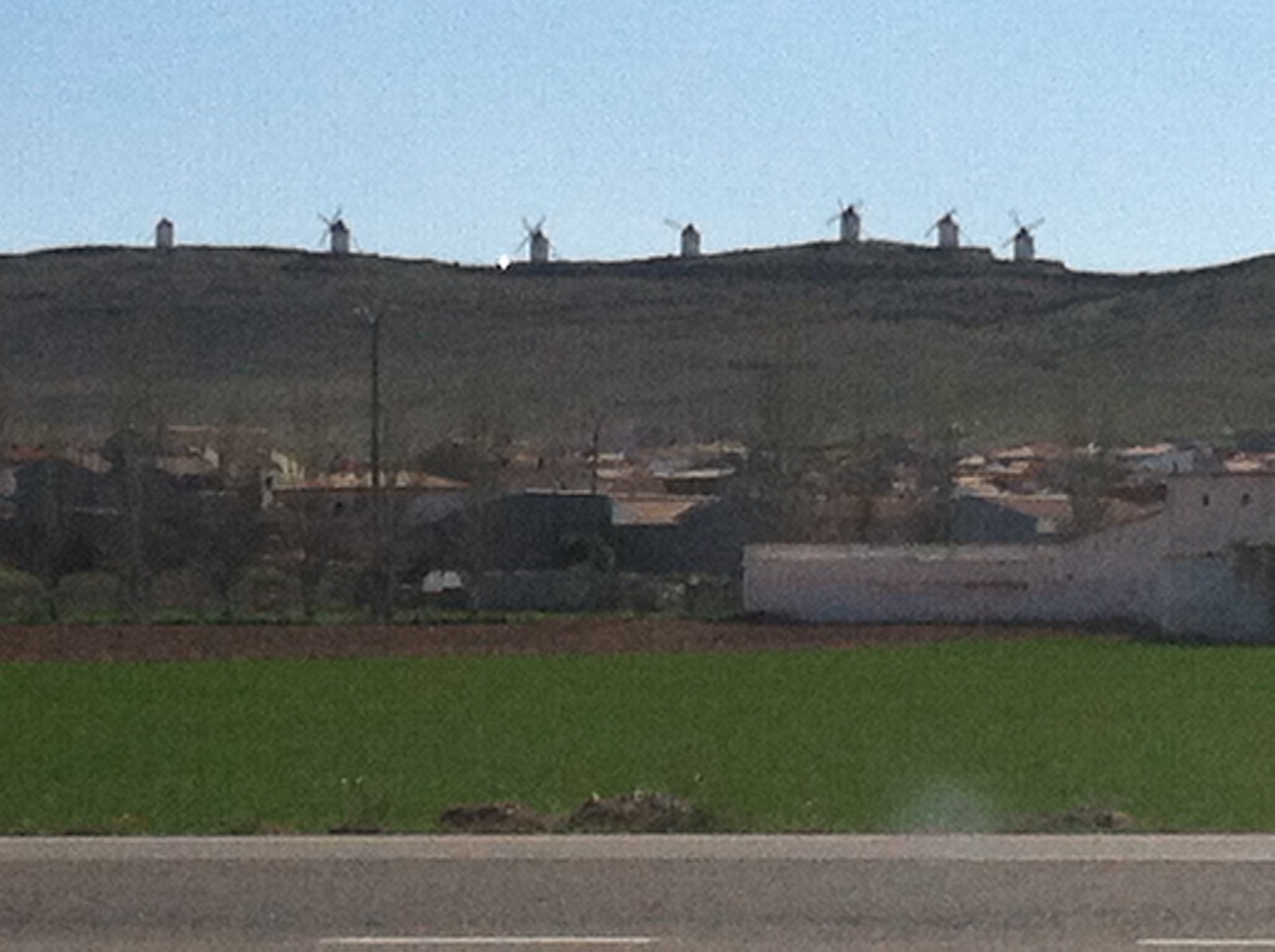In the image, a vibrant blue sky stretches across the background, providing a clear view of a gentle greenish-brown hill or ridge. Atop this hill stand seven white windmills, each with four blades and pointed black tips, their bases securely planted in the terrain. As the land slopes downward from the hill, a quaint village comes into view, characterized by light stone buildings with brown roofs. Interspersed among the buildings are leafless trees, suggesting the photograph was taken outside the blooming season.

Closer to the viewer, the details become more defined. Beyond the village, a lush, dark green field spans the width of the image, its appearance reminiscent of a baseball field with a patch of brown dirt possibly indicating an infield area. Adjacent to the field is a distinctive white building, enhancing the setting's picturesque quality. The foreground of the photograph is dominated by a gray asphalt road, punctuated by white dashed lines running horizontally. Despite the image's overall blur, the elements captured offer a serene and pastoral scene.